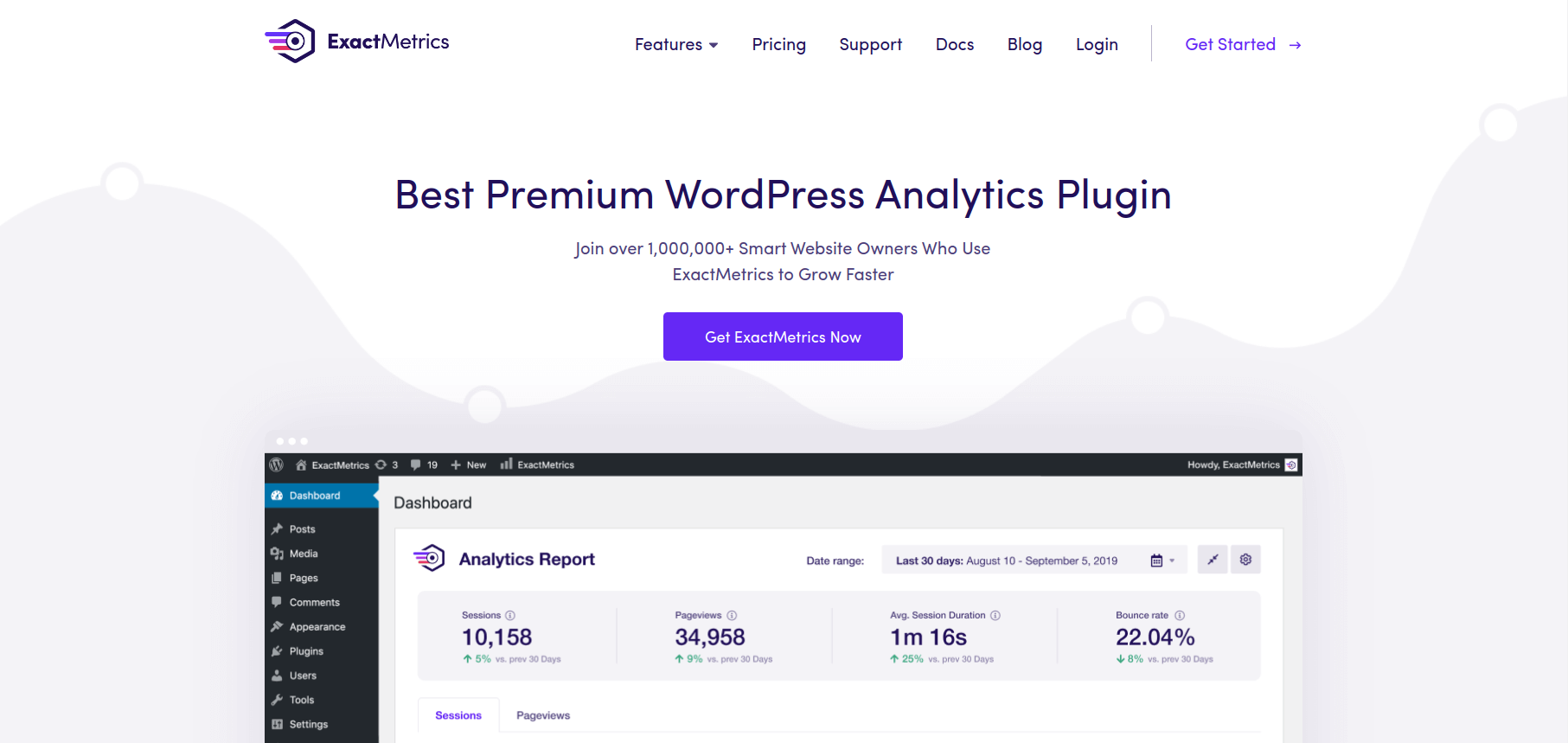The image is a detailed screenshot of the ExactMetrics business page, featuring its comprehensive analytics plugin for WordPress. In the top left corner, the ExactMetrics logo is prominently displayed, accompanied by a navigation bar that includes the options: Features (with a drop-down menu), Pricing, Support, Docs, Blogs, and Login. To the far right, there is a blue "Get Started" button with an arrow pointing to the right, suggesting it’s a clickable hyperlink.

Beneath the navigation bar, a bold headline reads, "Best Premium WordPress Analytics Plugin," inviting users to "Join over a million plus smart website owners who use ExactMetrics to grow faster." A blue box below this with white text reads, "Get ExactMetrics Now."

The main portion of the screenshot showcases an analytics report within a WordPress dashboard, identified by the recognizable 'W' icon in the top left corner and various navigation options listed vertically on the left sidebar. The sidebar includes: Dashboard (highlighted in blue), Posts, Media, Pages, Comments, Appearance, Plugins, Users, Tools, and Settings.

Central to the image is the Dashboard view, which displays the following analytics details under the "Analytics Report" section:
- **Date Range:** Last 30 Days, August 10th to September 5th, 2019
- **Sessions:** 10,158 (up 5% from the previous 30 days)
- **Page Views:** 34,958 (up 9% from the previous 30 days)
- **Average Session Duration:** 1 minute, 16 seconds (up 25% from the previous 30 days)
- **Bounce Rate:** 24.04% (down 8% from the previous 30 days)

These metrics highlight how ExactMetrics effectively provides detailed analytics for WordPress users, aiming to assist them in optimizing their website performance.

The entire image serves as a comprehensive example of how ExactMetrics functions, emphasizing its utility for those who use WordPress.